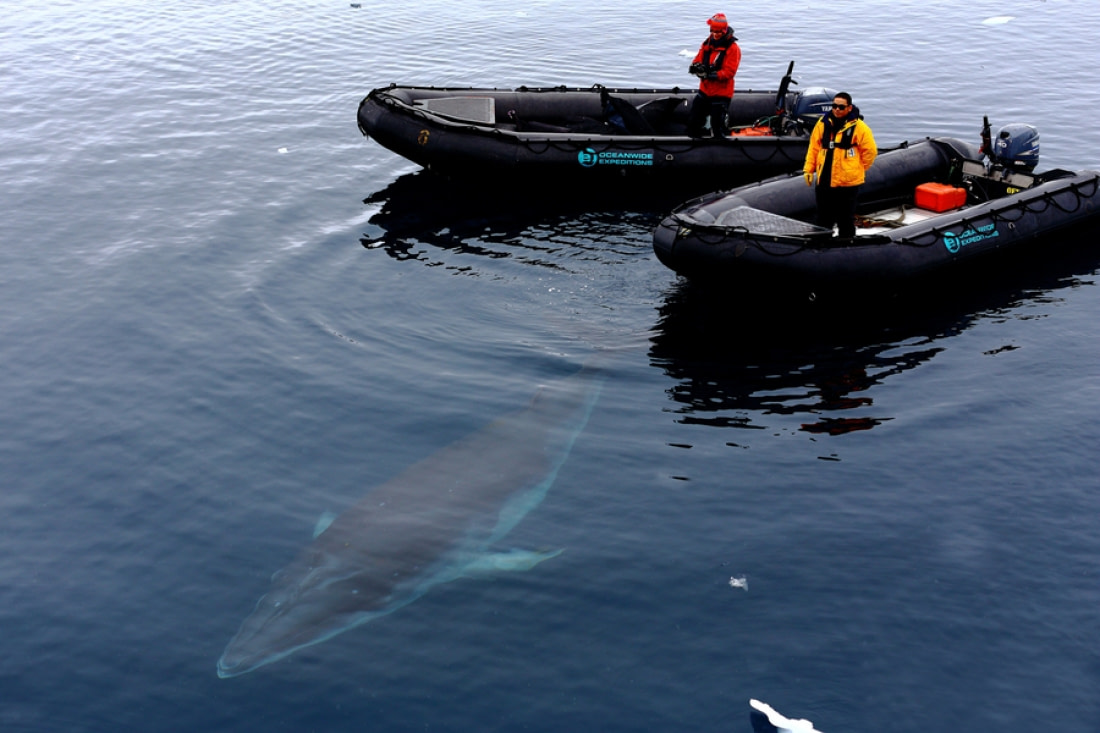In the image, there are two black speedboats in the ocean, both with blue text reading "Oceanwide Expeditions" accompanied by an icon. Each speedboat has a man onboard. The man on the speedboat centrally positioned at the top is dressed in a red life jacket, red hat, and black trousers. The man on the speedboat to the right is wearing a yellow life jacket, sunglasses, and black trousers; this boat also contains a red container. The water beneath the speedboats is rippling from their movement, and a whale, with a black top and light blue underside, is seen swimming towards the bottom left of the image. The scene is bathed in daylight, with sunlight reflecting off the water. The colors in the image include various shades of blue, grays, black, red, yellow, and light blue.